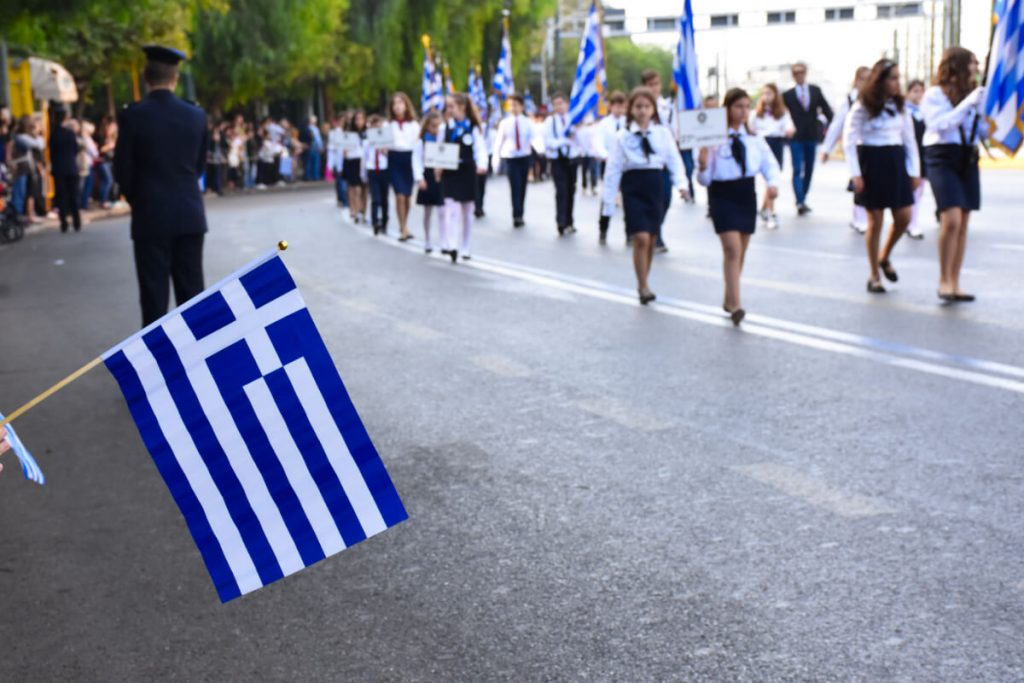The image depicts a bright, sunny day during a parade or march in Greece, evidenced by the numerous Greek flags, characterized by their white and blue stripes with a white and blue cross in the corner. The scene is filled with middle and high school-age children, predominantly girls clad in white shirts, dark blue skirts, matching dark ties, and dark shoes. The boys are similarly dressed in white shirts but with black slacks, sporting red or blue neckties. These students, approximately aged between 12 to 16 years, march in organized rows down the street, flanked by bystanders who line the roadside. Policemen are stationed to the side, ensuring order. Many onlookers wave small Greek flags, while in the background, tall green trees and a building provide a scenic backdrop. An adult, possibly a principal or teacher, walks alongside the students, donning a suit and blazer, overseeing the procession. The mood is festive and structured, underscored by the collective attire and national symbols.